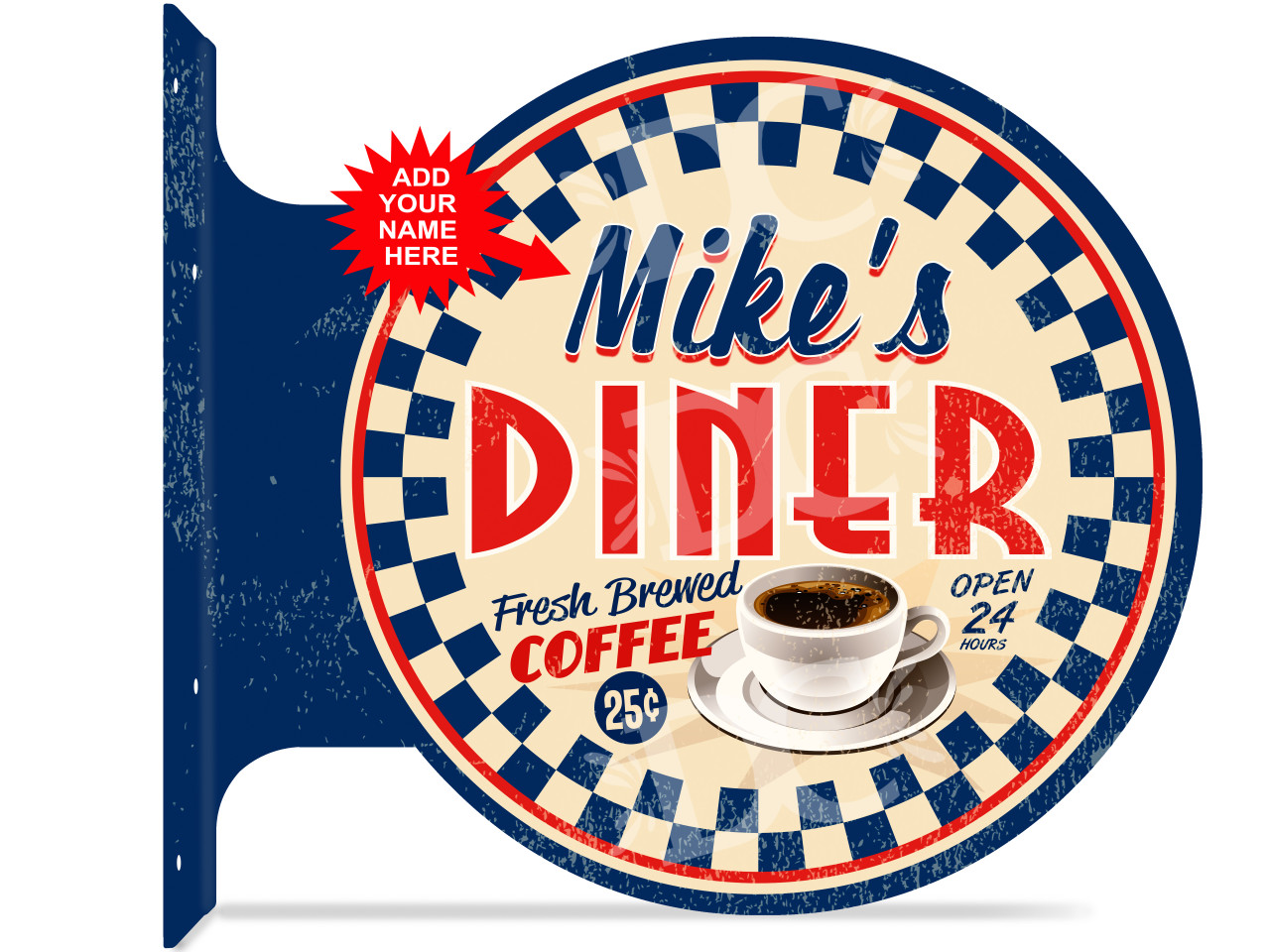The image features a vintage-style customizable diner sign with a predominantly white, whitish-gray background. The sign attaches to a post via a dark blue metal bracket on the left, which has four screw holes. The main round sign has a distinctive checkered border in blue and white, accentuated by red and white lines and a blue border. The top of the sign features a red sticker or arrow labeled "Add your name here," suggesting the sign's customizable nature. The text on the sign reads "Mike's Diner," with "Mike's" in blue and "Diner" in large red letters. Below this, on the left side, it advertises "Fresh Brewed Coffee, 25 cents" with an illustration of a coffee cup on a white saucer. To the right of the coffee illustration, within a circular area, it states "Open 24 Hours" in bold lettering. The detailed design elements and scuff marks give it an authentic, nostalgic diner aesthetic.